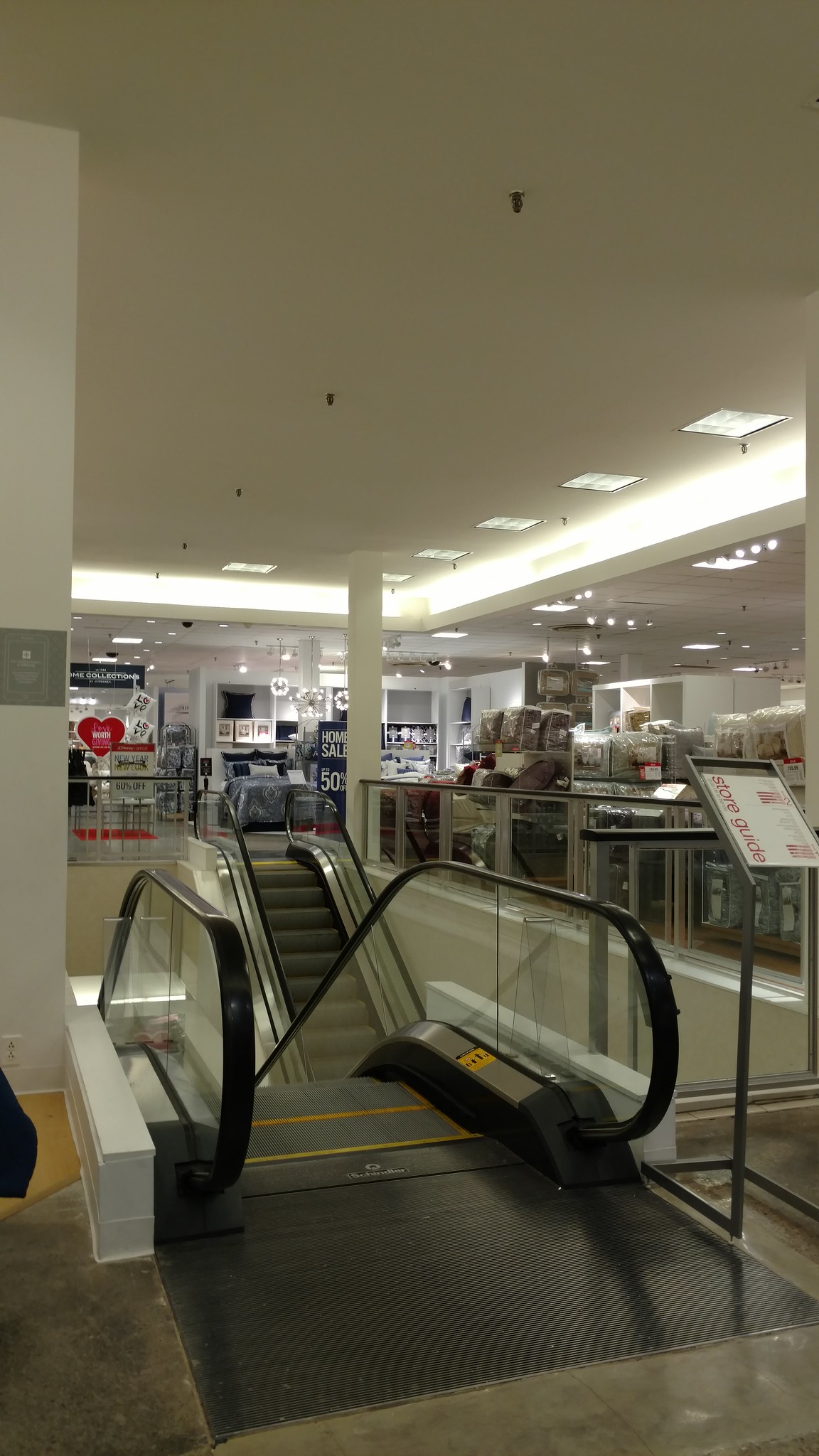The image showcases the interior of a bustling shopping mall or large supermarket, characterized by a pair of escalators centrally located within the frame. The escalator in the foreground appears to be descending, while the one in the background is out of focus but possibly ascending. Surrounding these escalators are neatly organized store displays, featuring an array of products stacked on white shelves and cases, particularly prominent on the right side of the image. The environment is well-lit, emphasizing the diverse assortment of merchandise available to shoppers. The scene captures a typical day within a commercial complex, highlighting both the functional architecture and the variety of goods on offer.